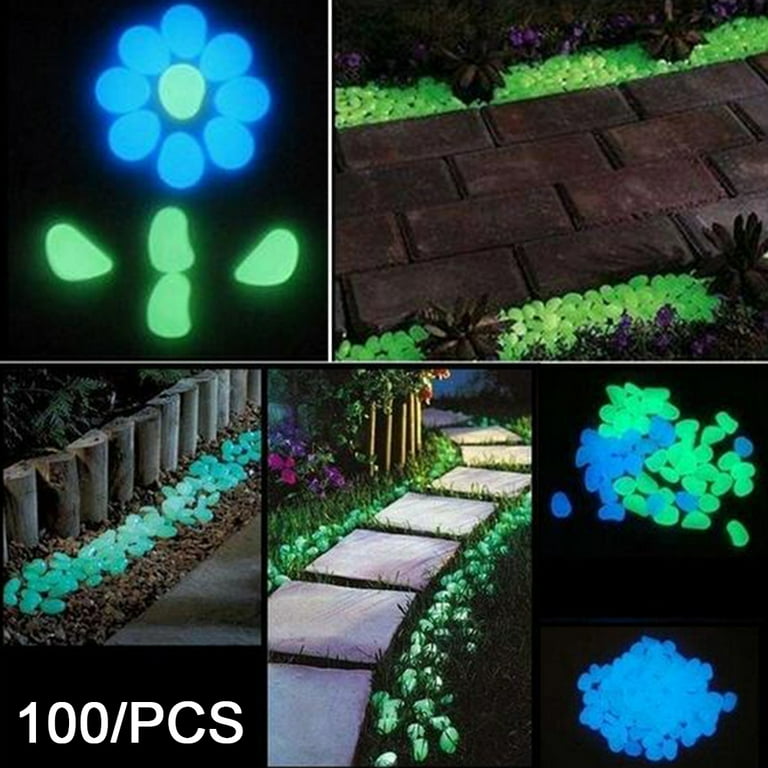The image depicts the outside packaging of a product containing 100 glow-in-the-dark pebbles, illustrated in vivid detail. In the bottom left corner, a black rectangle with white text clearly states “100 / PCS,” indicating the quantity included. The main visual is a large square composed of five smaller rectangles, each showcasing different uses for the pebbles. The upper left pane features a glowing blue flower with a neon green stem, intricately depicted with concentric circles. To its right, a brick sidewalk is adorned with bright green floral designs along the edges, enhancing its aesthetic appeal. The lower left pane displays lime green stones scattered amid brown rocks along a walkway. In the center bottom image, square stepping stones are flanked by bright green balls amidst grassy surroundings. The lower right pane shows small piles of phosphorescent blue and green pebbles, vividly glowing in the dark. These images collectively highlight various creative and decorative applications of the pebbles, making them a versatile and visually appealing product for beautifying outdoor spaces.